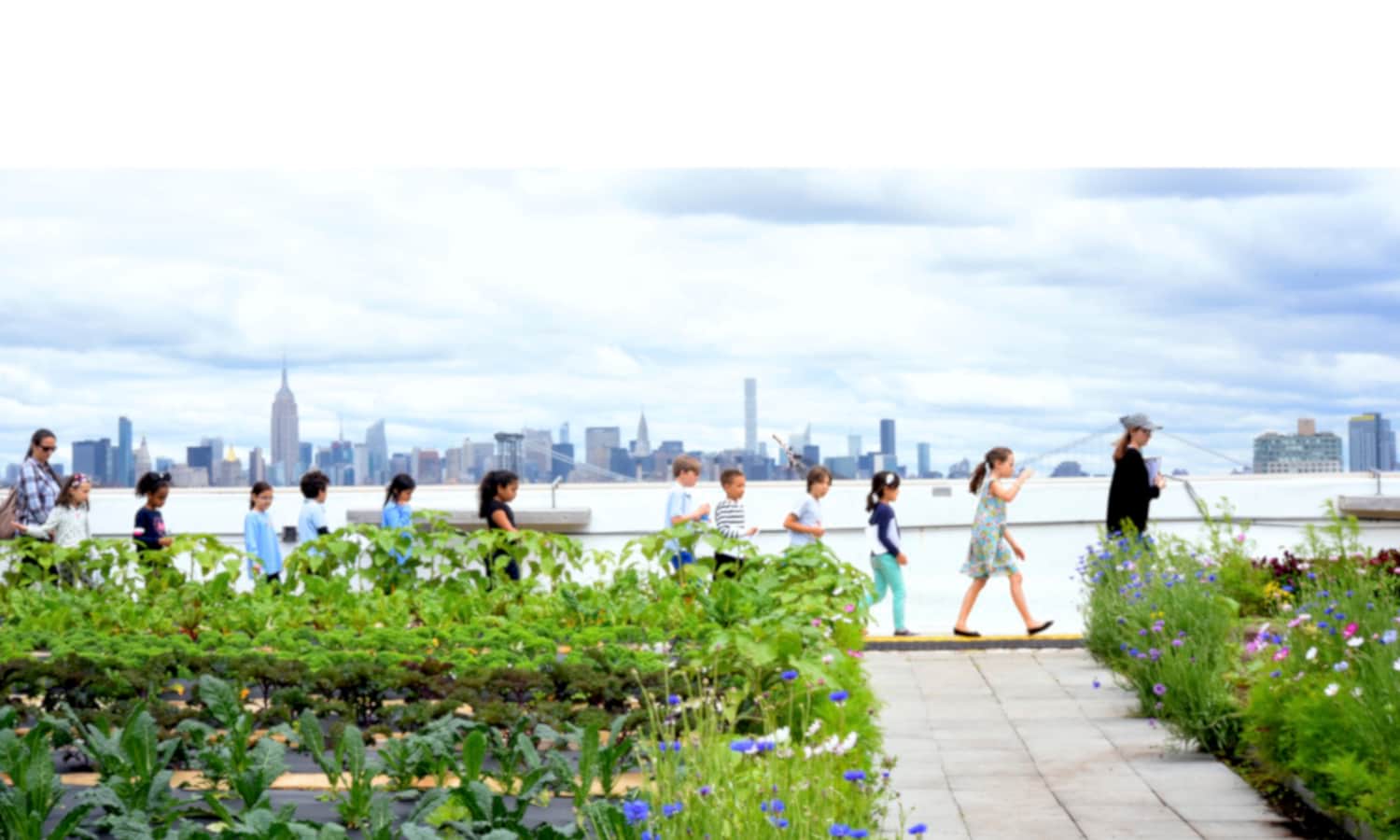The image captures a vibrant, outdoor scene featuring a diverse and colorful flower garden in the foreground. The garden is alive with blue, white, red, pink, and yellow blossoms, as well as large green leaves, possibly from vegetable plants, particularly in the lower left corner. Amongst the flowers, ferns, and shrubs, a group of ten young students, possibly aged between 7 and 9, along with what seem to be their teachers or chaperones, are walking from left to right across a brick sidewalk. Leading the group is a woman dressed in a black sweater and a gray hat, followed by a young girl in a blue dress with a ponytail, and several other children in various colorful outfits including jerseys, slacks, t-shirts, and dresses.

Towards the back of the line, another adult, possibly also a teacher, wearing a checkered blouse and sunglasses, brings up the rear. In the distance, beyond the garden, a significant city skyline is visible, filled with numerous buildings and skyscrapers, including a structure resembling the World Trade Center. Above, blue and white clouds scatter across the sky, enhancing the lively and bustling atmosphere of the scene. The body of water, hinted at behind the children, supports boats and docks, adding another layer of depth and activity to the image. Overall, it appears to be a class outing or an educational walk against the picturesque backdrop of what could be New York City.